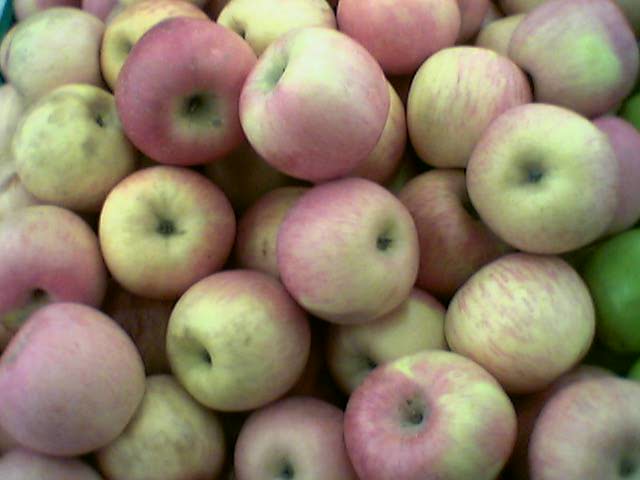The photograph showcases a large pile of apples, completely covering the frame with no visible background. The apples vary in color, predominantly displaying muted shades of yellow, green, and pinkish-red, rather than the expected bright reds and greens. Most apples exhibit a dull, lackluster appearance, possibly unprocessed, with no shine to their skin. Among the apples, there are distinct patches: some apples are more green, some are a mix of green and pink, and a few are almost entirely pink. Off to the right side, a cluster of solid green apples, possibly bruised, adds to the variety. The apples are tightly packed together, creating a layered effect from corner to corner and side to side, resembling a bountiful harvest at a fruit stand.